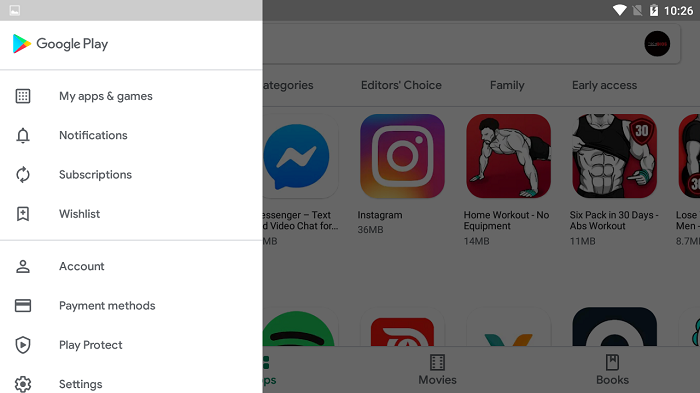In this photograph, a person is browsing the Google Play Store on what appears to be a tablet or possibly a laptop with a small window. The interface is divided into two main sections with an open slider panel on the left-hand side. The Google Play triangular logo is prominently displayed in the upper left corner next to the text "Google Play."

Below this logo, a vertical menu is presented, including various sections such as "My apps & games," "Notifications," "Subscriptions," "Wishlist," and a grey bar separating subsequent options like "Account," "Payment methods," "Play Protect," and "Settings." 

Occupying approximately 65% of the image on the right side, we see a greyed-out background beneath which several app categories and representative apps are visible. The categories listed include "Categories," "Editor's Choice," "Family," and "Early Access." Featured apps such as a messenger app, Instagram, a home workout app, and a six-pack workout app are clearly identifiable. Although some additional apps and categories are visible at the bottom, they are partially cut off from the view.